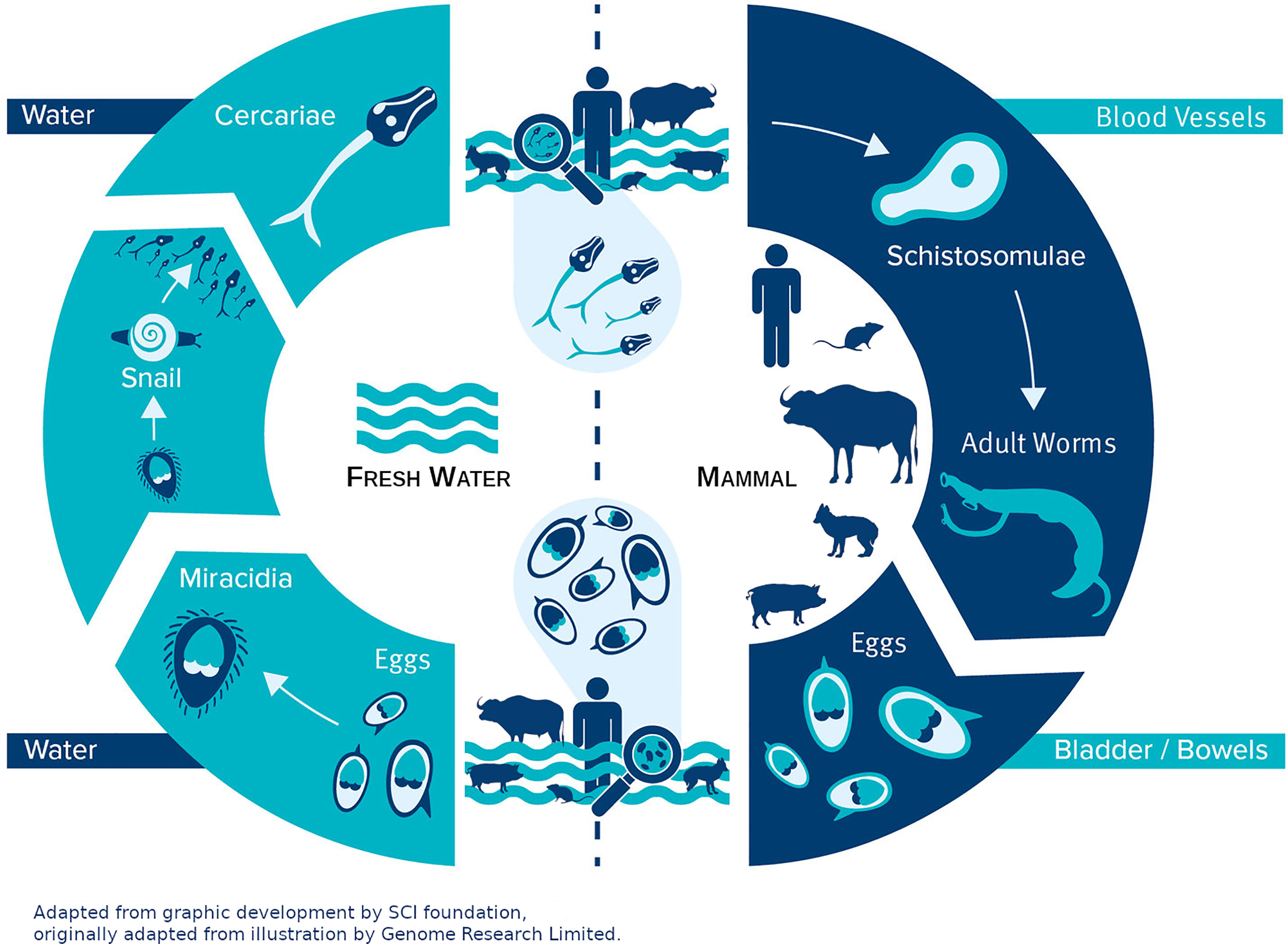This highly detailed graphic, originally developed by SCI Foundation and adapted from an illustration by Genome Research Limited, presents a complex circular diagram related to the life cycle of schistosomes. The diagram is divided into two half-circles—one darker blue on the right, representing blood vessels and water and bowels, and the other lighter blue on the left, signifying fresh water and various stages of life forms.

The outer sections of the circle feature technical terms and horizontal rectangular labels such as "blood vessels," "water," and "bowels," associated with specific points in the life cycle. The diagram follows a cyclical flow, marked by arrows that lead from one stage to the next.

Inside the circle, detailed illustrations depict the involvement of humans, mammals (including cows, pigs, and rats), and various stages of microorganisms such as adult worms, schistosomes, eggs, miracidia, and a snail. Particularly notable are segments illustrating process stages: the development from eggs to miracidia, and the transition from snails to another life stage called cercaria.

A stick figure with a magnifying glass at the top of the diagram symbolizes closer examination of this life cycle. The design is filled with blue tones, and wavy lines emphasize the water element in the cycle, with sections depicting waves in the bottom middle and top middle. The graphic is a comprehensive depiction of the interconnectedness between water, blood vessels, and various organisms, elucidating the schistosome life cycle.